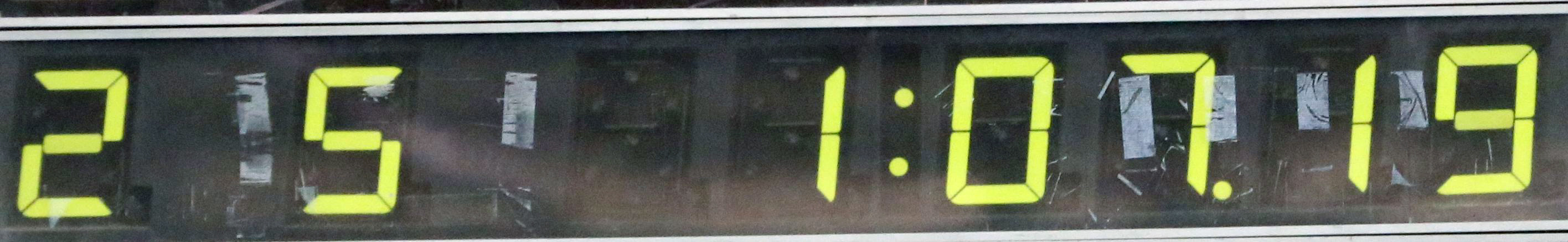The image depicts a weathered, long rectangular timekeeping device, possibly an odometer or alarm clock, with a primarily black background. It features 8 slots for displaying numbers, framed by square outlines. The numbers displayed are in a light greenish-yellow hue: '2', followed by '5', an empty slot, '1 dot dot 07 period', and '19'. At the top, there are two strips of gray metal. The numbers are likely indicators of time, suggesting it might be tracking 1 hour, 7 minutes, and 19 seconds.